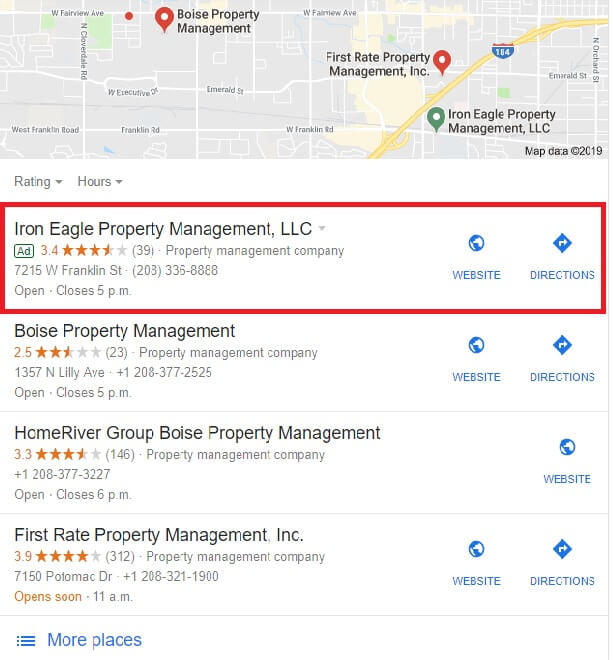A screenshot from a 2019 website shows a detailed map with several property management companies pinned. Prominently featuring Highway 184, the map includes locations such as Boise Property Management, First Rate Property Management, Inc., and Iron Eagle Property Management, LLC. Below the map is a section labeled "Rating and Hours," highlighting search results for these companies. Iron Eagle Property Management, LLC, bordered in red as an ad, has a rating of 3.4 stars, and provides links to its website and driving directions. Boise Property Management has a 2.5-star rating with similar links. Home River Group Boise Property Management earns 3.3 stars and offers a website link but lacks directions. The highest-rated, First Rate Property Management, boasts 3.9 stars.